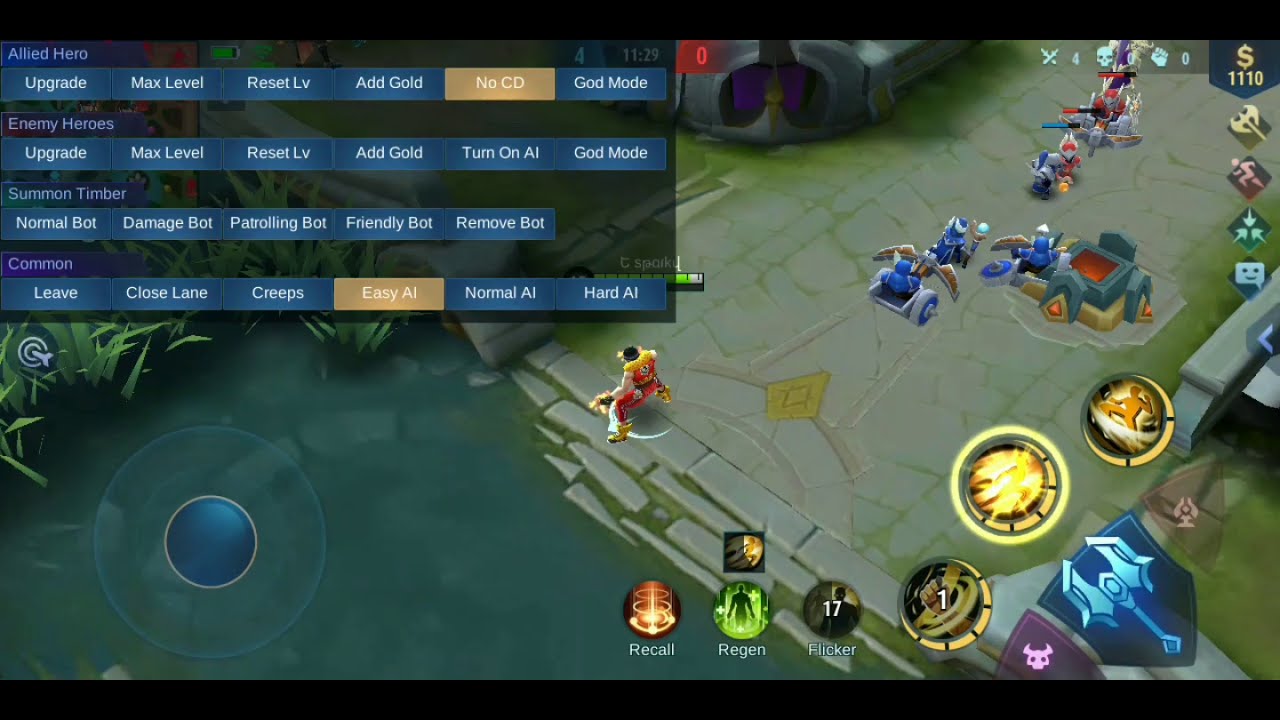The image is a screenshot of a video game depicted in a top-down view with a cartoonish design. The environment resembles a forest area featuring pavement made of old stone interspersed with moss and a shallow creek to the left. In the upper left quadrant of the screen, there's an interface with blue boxes housing white text, presenting numerous options including "Allied Hero," "Enemy Heroes," "Summon," "Upgrade," "Max Level," "Reset Level," "Add Goal," "Turn on AI," and various bot commands like "Normal Bot," "Damage Bot," and "Friendly Bot." The bottom left corner features concentric circles, while the right half of the image showcases NPCs and different avatars. Circular logo icons populate the lower right quadrant, and the upper right quadrant displays a dollar sign with the amount 1110 and four icons beneath it. The game seems to blend basketball elements with vehicular gameplay, highlighted by green and gold buttons labeled with options like "Closed Lane," "Maximum Level," and "Reset Level."